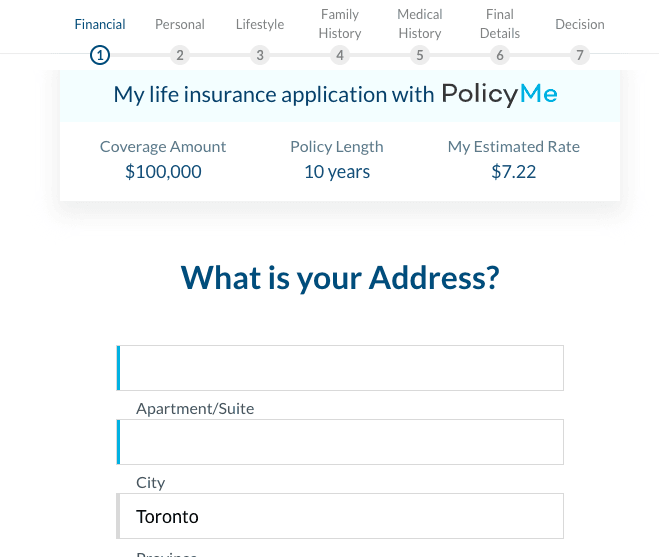This image depicts a smartphone screen displaying a life insurance application from Policy Me. At the top of the screen, there is the word "Financial" with a circled number "1" in blue beneath it. Subsequent columns labeled "2" through "7" appear in gray, each topped with specific categories: "Personal," "Lifestyle," "Family History," "Medical History," "Final Details," and "Decision."

The header of the application reads, "My Life Insurance Application with Policy Me," with "me" highlighted in blue. Displayed below are the coverage details: a coverage amount of $100,000 and a policy length of 10 years, with an estimated rate of $7.22. 

A section prompts for the user's address, featuring input fields marked by faint blue slivers on the left side. One of these fields, designated for the city, has "Toronto" already typed in. Additional fields are provided for the user's physical address and apartment or suite number.